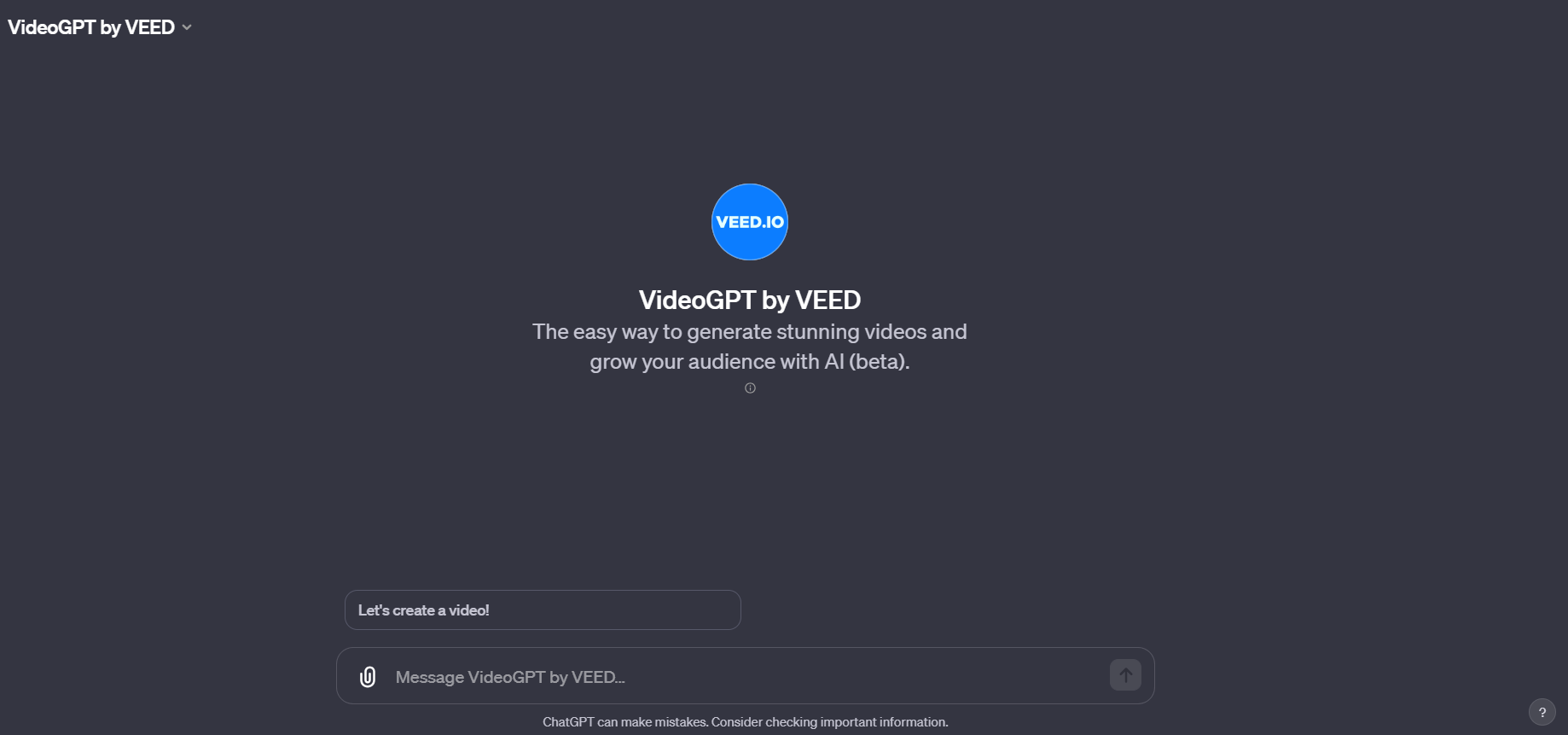This image depicts a video GPT webpage with a predominantly black background and a large, central square. The top-left corner of the square features the text "Video GPT by V," with the "V" being in a capital letter (V-E-D). 

In the center of the image rests a prominent blue circle, inside of which are the characters "V . I-O." Beneath this, the text reads: "Video GPT by V. The easy way to generate stunning videos and grow your audience with AI." The word "beta" appears in parentheses, denoting the version of the service.

Below this central section, and slightly to the left, are two rounded rectangular buttons. The first button reads "Let's Create a Video," while the second button says "Message Video GPT by V," followed by an ellipsis. Adjacent to the word "Message," there is a paper clip icon, and to the far right of this button, there is an upward arrow icon.

At the bottom of the image, there's a disclaimer stating: "Chat GPT can make mistakes. Consider checking important information." In the very bottom right corner, a question mark icon is present, presumably serving as a help or support option.